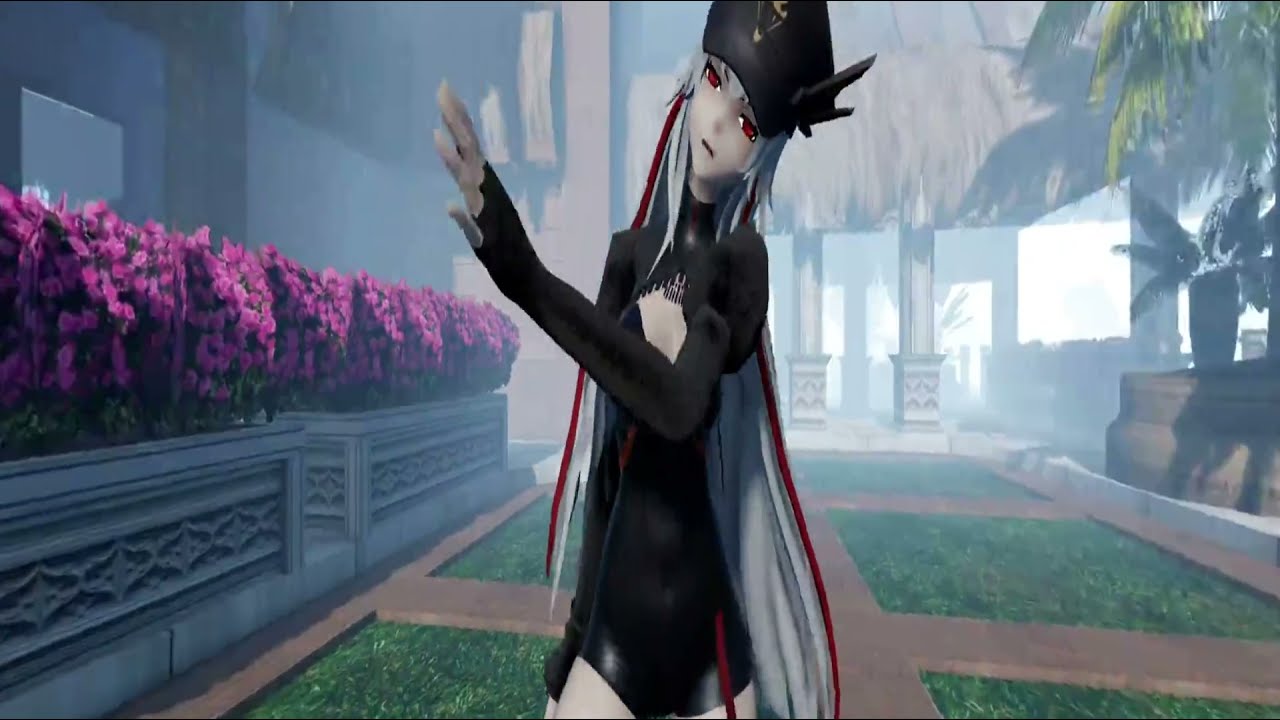The image appears to be a detailed and captivating screenshot, potentially from a video game or an anime, showcasing a young female character. The character is centrally positioned and facing the viewer, embodying a striking appearance with long flowing gray hair that extends to her thighs, accented with red streaks. Her eyes are a vivid, vampiric red, enhancing her mysterious presence.

She dons a black, high-collared bodysuit made of a leather-like material, which features a V-neck inset revealing part of her chest. Complementing her outfit, she wears a distinctive black pirate-style hat. Adding a splash of color to her ensemble, a red cape with a gray lining drapes over her shoulders.

The setting is a misty or foggy garden, contributing to the magical or mysterious ambiance of the scene. The ground beneath her consists of a paved surface in a grid-like pattern with squares of green grass. To her left, there are gray concrete planters filled with purple flowers, while to her right, brown planters house a palm or banana tree, alongside another smaller tree. This blend of floral elements and planned greenery enhances the fantastical feel of the environment, making the character stand out as an intriguing figure within this mystical garden.